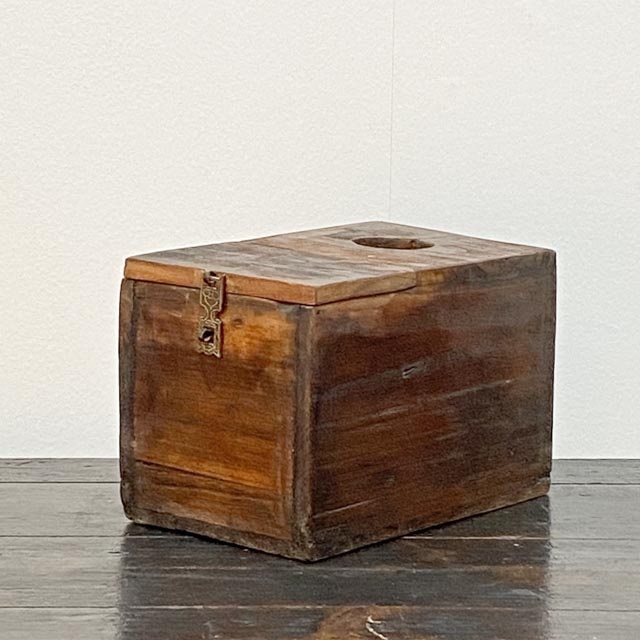The image depicts a rustic, brown wooden crate resting diagonally on a dark-stained, varnished wooden floor, set against a light tan or beige background. The crate, composed of horizontal wooden slats, features varying shades of brown, giving it an aged and weathered appearance. A brassy, brownish-gold latch is attached to the middle of the left side of the crate, designed with a square cutout at the bottom where it latches onto the lid. The lid of the crate has a circular hole on the right-hand side, approximately two and a half inches in diameter. This circular cutout stands out against the otherwise solid wooden surface of the crate.